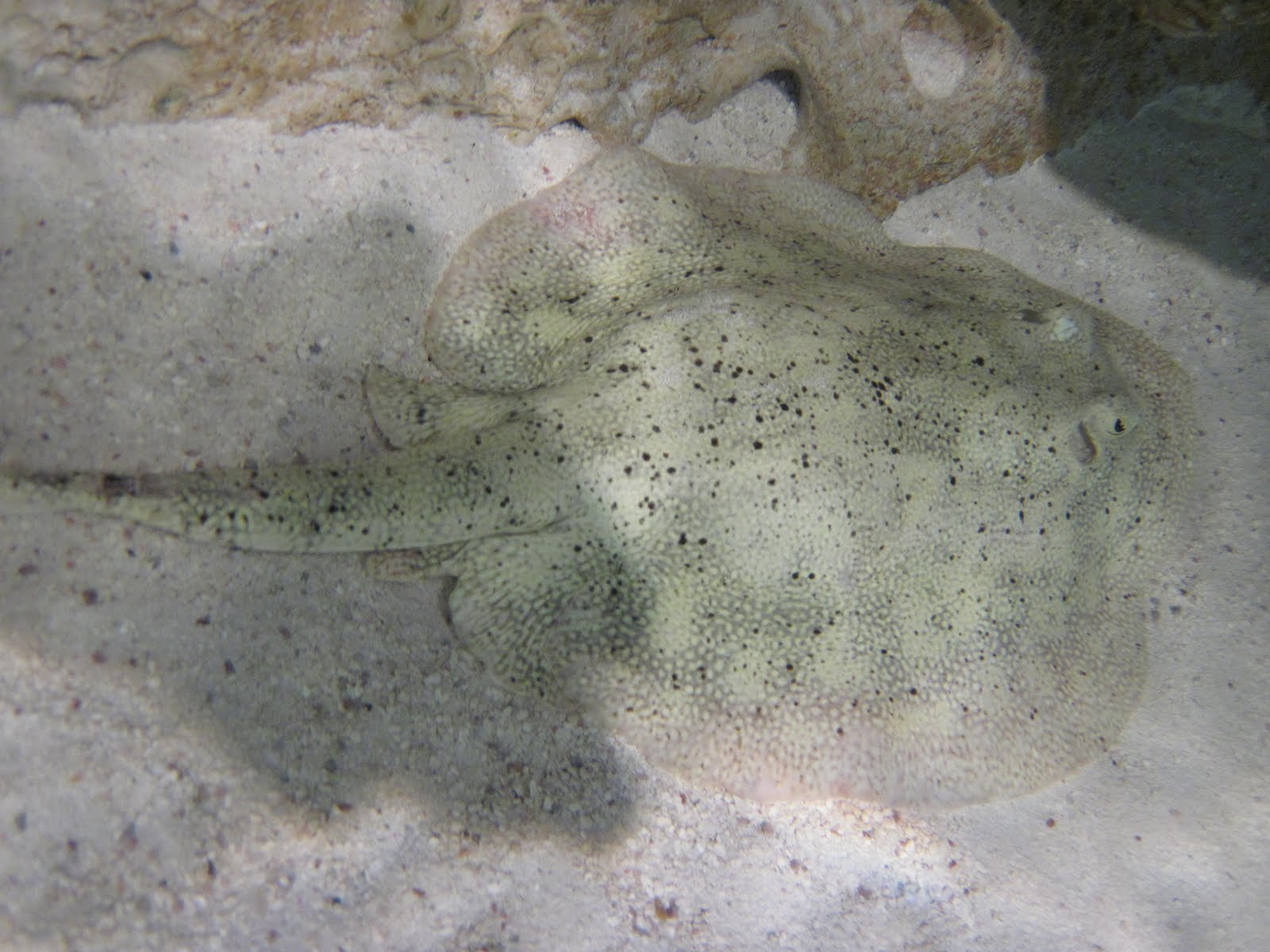In this underwater image, a stingray is seen resting on the seabed floor. The stingray exhibits a milky color with pinkish sides and features distinct black speckles across its body. Its eyes are positioned on top of its head, and the tail, situated to the left side of the picture, showcases the same speckled pattern. The seabed consists of coarse, whitish sand interspersed with brown spots and white rocks. In the upper part of the image, a brown, rocky structure resembling a coral reef is visible, which appears somewhat dusty. The stingray blends seamlessly with its surroundings due to its camouflage coloring, which mirrors the seabed and surrounding environment. Shadows are cast at the top right corner of the image, adding depth to the scene.